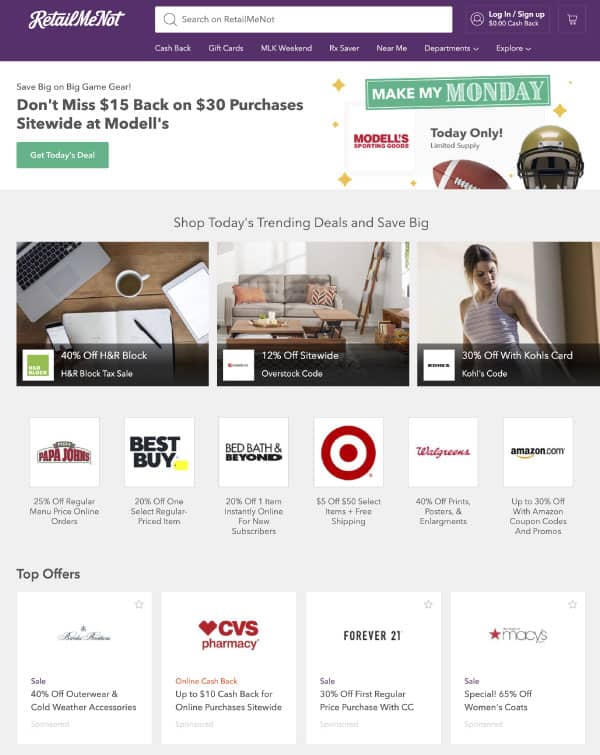**Detailed Caption for RetailMeNot Web Page Image**

The featured image displays the RetailMeNot homepage, characterized by a distinctive dark purple background. Centered at the top is the RetailMeNot logo in a cursive font. Below the logo is a prominently placed search bar, featuring a magnifying glass icon followed by the text "Search on RetailMeNot." 

On the right side of the header, a silhouette icon is accompanied by the bold white text "Login/Sign Up." Nearby, another text in white reads "$0.00 Cash Back." Additionally, there is an icon of a shopping cart, also on the right.

Beneath these elements, a row of clickable buttons is arranged horizontally, labeled: “Cash Back,” “Gift Cards,” “MLK Weekend,” “Rx Saver for Prescriptions,” “Near Me,” “Departments,” and “Explore.” Each button indicates dropdown menus with a down arrow symbol.

Adjacent to these buttons, within a white section on the left side, a promotional banner says “Save Big on Game Gear.” Below this, in bold black font, it states, “Don't miss $15 back on $30 purchase sitewide at Modell's” with an additional emphasis on “M-O-D-E-L-L”. Further down, there is a teal or dark green button that says “Get Today’s Deal” in bold white text.

To the right of this promotional content, there's a section with diamonds and the text “Make My Monday,” followed by “Modell’s Sporting Goods” in red. Adjacent in bold black text, it says, “Today Only.” Below this message, the text indicates a limit applies. The same section displays a brown football with white stripes and stitching, alongside a tan football helmet with a black faceplate and white interior.

Below this primary promotion area is a dark gray rectangle containing black text, stating, “Shop Today’s Trending Deals and Save Big.” To the left, an illustration features a meeting area with a table, a gray laptop with black keys, an open book with a pen, a person holding a cell phone, and a white tablet. The cell phone has a black bezel.

Further down the page, the "H&R Block" logo is displayed within a green square. The adjacent offer highlights "40% off H&R Block Tax Sale." Another promotion features a gray loveseat with one orange and one red-striped cushion, advertising "12% off sitewide Overstock code."

A fit woman with short hair, wearing a sleeveless tank top with purple stripes, is depicted looking down towards the right, indicating a "30% off Kohl’s Card" offer.

The footer of the page lists major retailers such as Papa John’s, Best Buy, Bed Bath & Beyond, Target, Walgreens, and Amazon within a gray background area. The top offers include “40% off Outdoor and Cold Weather Accessories” from CVS Pharmacy, “Up to 10% Cash Back for Online Purchases Sitewide.” Additionally, “Forever 21 Sale 30% off Regular Price Purchase with Credit Card,” and “Macy’s Sale Special 65% off Women's Coats” are mentioned.

This detailed description captures the essence and layout of the RetailMeNot homepage as seen in the image.